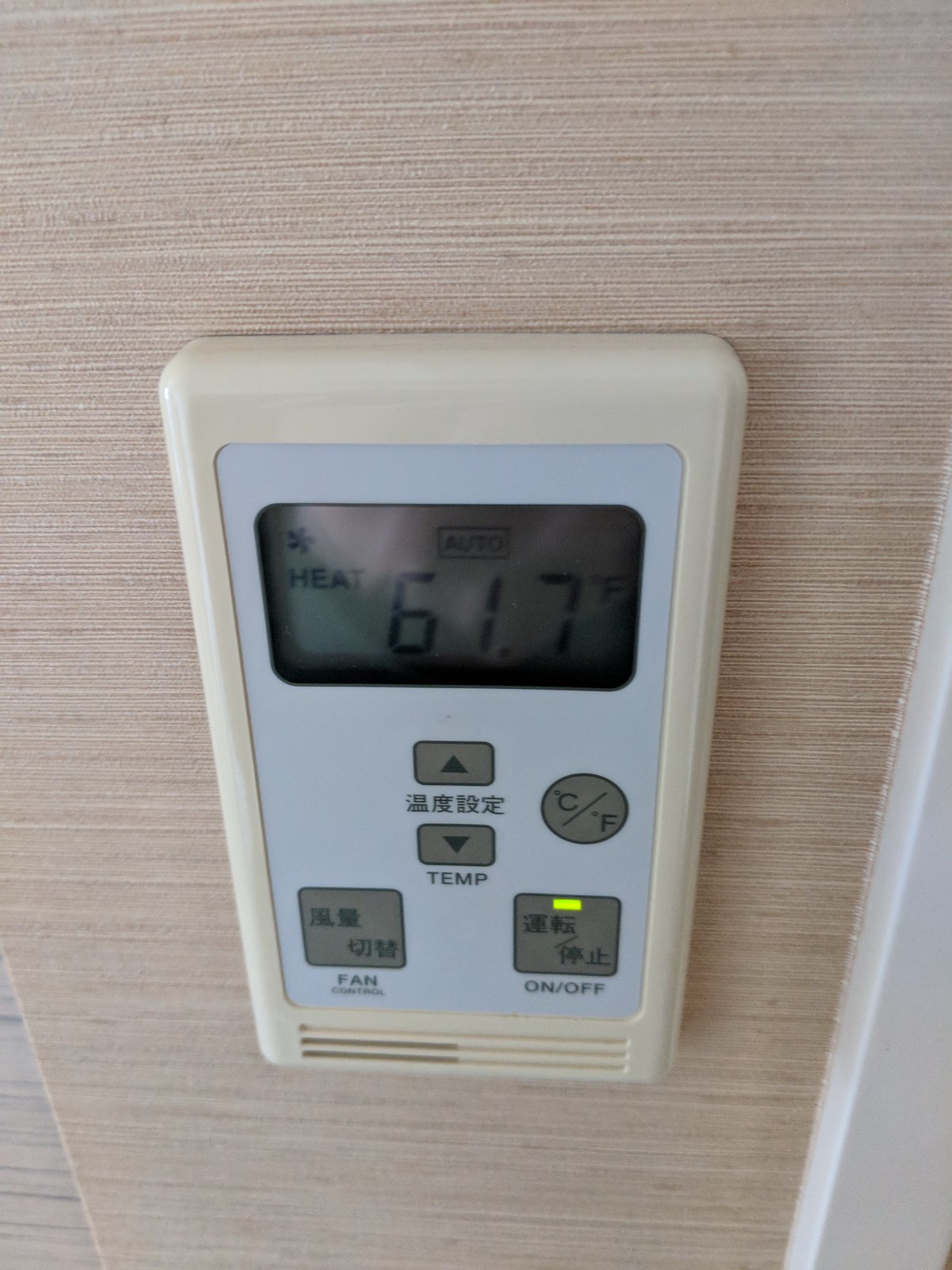In the center of the image, we see a thermostat mounted on a wall. The thermostat's outer casing is a light gray plastic, while its inner display area features a grayish-blue hue. The unit is affixed to a light brown wall, which is decorated with horizontal stripes, giving it a wooden-like texture. 

The surrounding wall fills most of the image, extending from the top to the bottom, but both the bottom right and bottom left corners reveal different adjacent walls. The bottom right corner shows a solid white painted wall. In contrast, the bottom left corner exposes a grayish wall adorned with black horizontal stripes.

Focusing back on the thermostat, it has distinct control features: a central button flanked by an up arrow above and a down arrow below, with the word "temp" underneath the down arrow. Additionally, there are two square buttons: one on the bottom left labeled "fan" and the other on the bottom right labeled "on/off." At the top center of the thermostat's display, there is a small window that reads "heat" with a temperature indication of "61.7 degrees Fahrenheit" and the word "auto" positioned above this display.